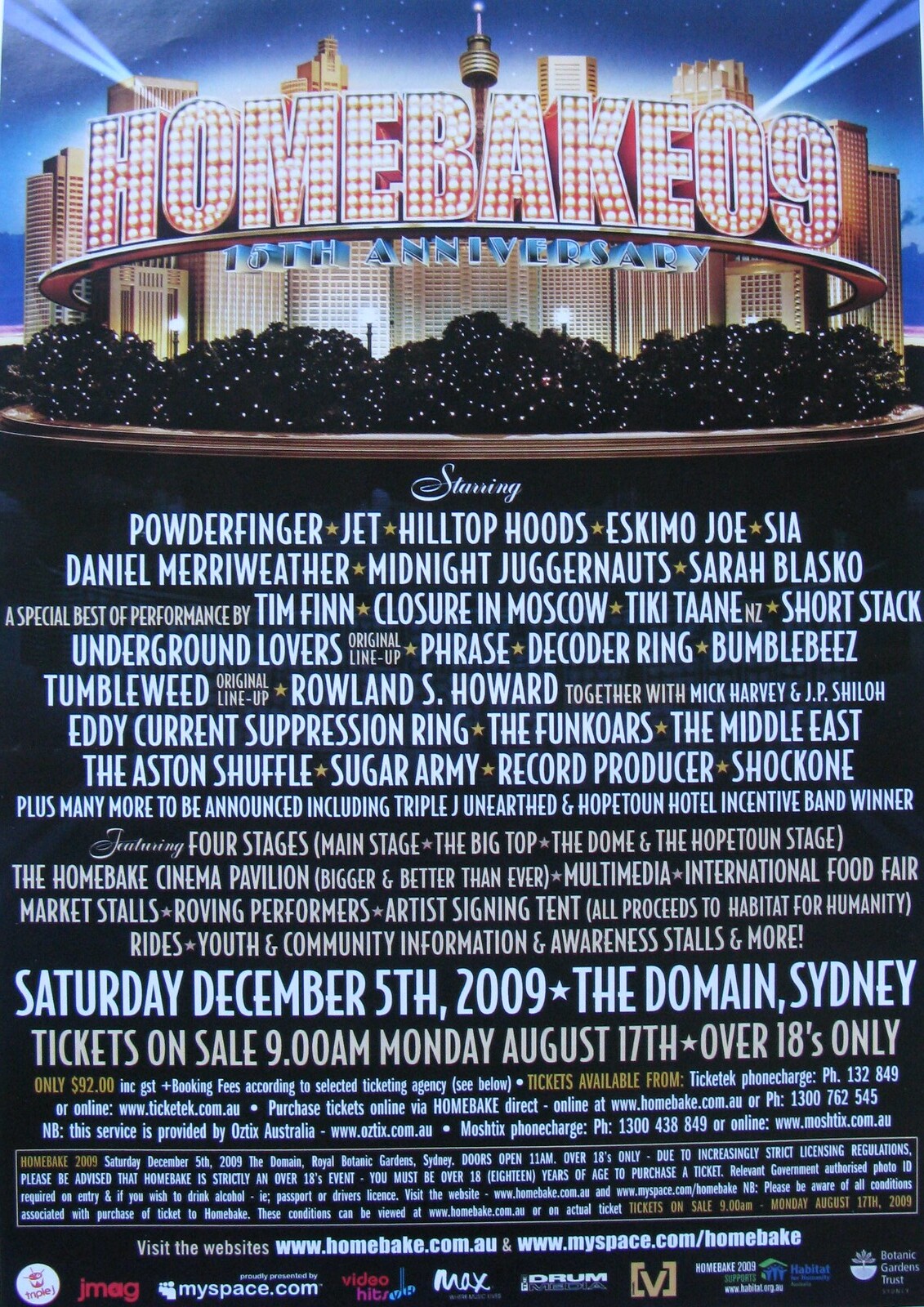The image is a detailed flyer for "Home Bake 09," celebrating its 15th anniversary. Set against a backdrop that resembles a night sky with a cityscape, likely Sydney, highlighted by spotlights and streetlights. The event's title, "Home Bake 09 15th Anniversary," shines brightly in glittering lights at the top. Featuring a stacked lineup of performers, the flyer lists Powderfinger, Jet, Hilltop Hoods, Eskimo Joe, Sia, Daniel Merriweather, Phrase, Decoder Ring, Bumblebees, Tumbleweed, and The Ashton Shuffle, with promises of additional acts to be announced. Important event details, including the date—Saturday, December 5th, 2009—and venue, The Domain in Sydney, are prominently noted. Tickets, going on sale at 9 am Monday, August 17th, require attendees to be over 18, with purchase options and more event specifics, such as supporting acts like Triple J, available on websites www.homebake.com.au and www.myspace.com/homebake. The flyer also mentions various attractions like multimedia displays, food fairs, market stalls, performances, and artist signings, all supporting Habitat for Humanity Australia. The bottom includes logos and sponsors, reinforcing the festival's grandeur and festivities.